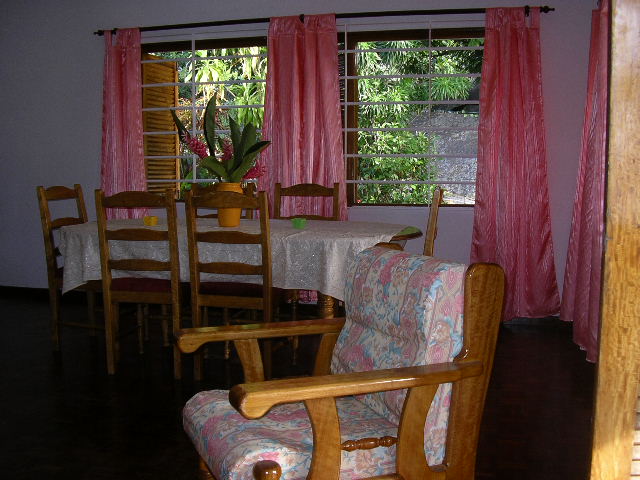The image is a color photograph depicting the interior of a house, specifically a dining room. Central to the scene is a wooden dining table adorned with a white tablecloth, surrounded by six wooden chairs—two on each side and one at each end. The table is positioned against a backdrop of two large windows draped with long pink curtains hanging from a dark curtain rod. The windows, framed in white and possibly featuring iron bars or wooden frames, provide a view of lush, tropical greenery outside, indicating a warm, sunny day.

In the background, on the dining table, there is a yellow flower pot containing a large, leafy green plant. In the foreground, there is a smaller, padded sitting chair facing away from the table, suggesting it might be oriented towards a TV or another focal point in the room. The chair's upholstery features a white and pink pattern, and its wood matches the dining table and chairs, creating a cohesive look within the room. 

Overall, the combination of the tropical outdoor scenery and the detailed interior furnishings suggests a warm, inviting atmosphere.